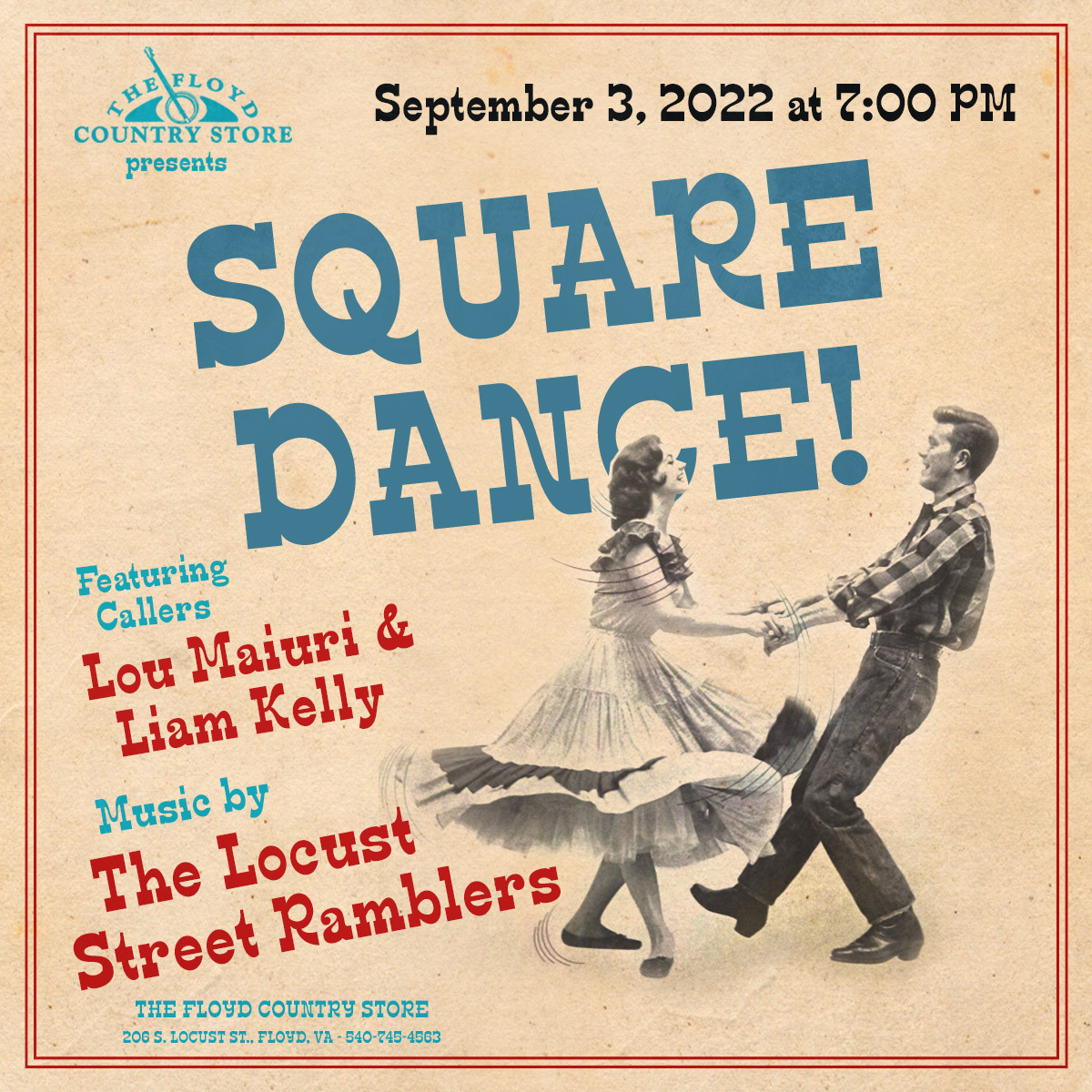This is a detailed square ad or flyer for a square dance event. The poster features an old-timey design with a browned, yellowed paper background, accented with red and blue elements reminiscent of a country store aesthetic. The headline reads "Square Dance!" in big blue letters, with "The Floyd Country Store Presents" in the top left corner. The event is scheduled for September 3, 2022, at 7 p.m. The advertisement highlights that the evening will feature callers Lou Maiuri and Liam Kelly, accompanied by music from the Locust Street Ramblers.

The left side of the flyer lists the details in various fonts and colors: "Featuring Callers" in blue, "Lou Maiuri and Liam Kelly" in red, "Music By" in blue, and "The Locust Street Ramblers" in red. The location is specified as 206 South Locust Street, Floyd, VA, with a contact number 540-745-4563.

An image centered to the right portrays a joyful scene of a white woman and a man square dancing. The woman, wearing a flowy, frilly dress that twirls as she dances, holds her hands out with a smile aimed at her partner. The man, clad in a checkered plaid shirt, jeans, and cowboy boots, leans back on his heels, his front leg kicked up in a lively dance move. This vibrant and nostalgic artwork effectively captures the lively spirit and traditional charm of the square dance event.